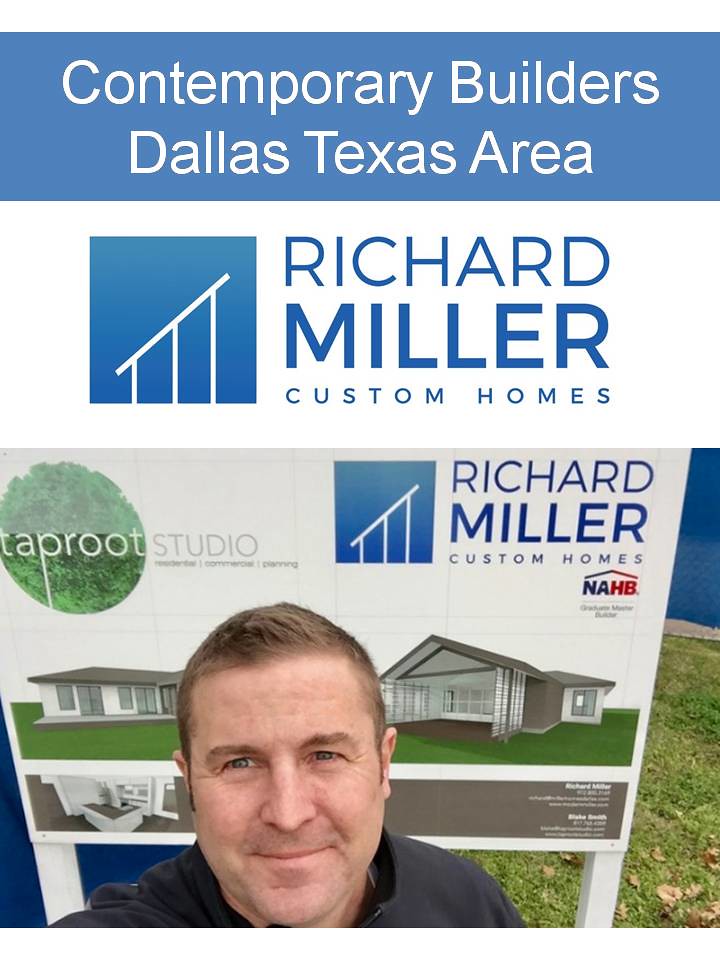The image features a white gentleman with short light brown hair, smiling and looking directly at the camera. He appears to be taking a selfie from an upward angle, capturing himself from the chin up. The background prominently displays a realtor sign that advertises Richard Miller Custom Homes, a member of the National Association of Home Builders (NAHB). The sign, produced by Tap Root Studio, is visually appealing with a contemporary design featuring medium blue borders and white printing. It reads "Contemporary Builders, Dallas, Texas area" at the top in white on a blue banner. Below this banner, the sign has a small square logo resembling the outline of a house, accompanied by the text "Richard Miller Custom Homes" in blue on a white background. The sign also includes a computer-generated image of a modern home and additional text that is not clearly legible. The ground beneath the sign shows some grass and dead leaves, adding a touch of natural context to the setting.